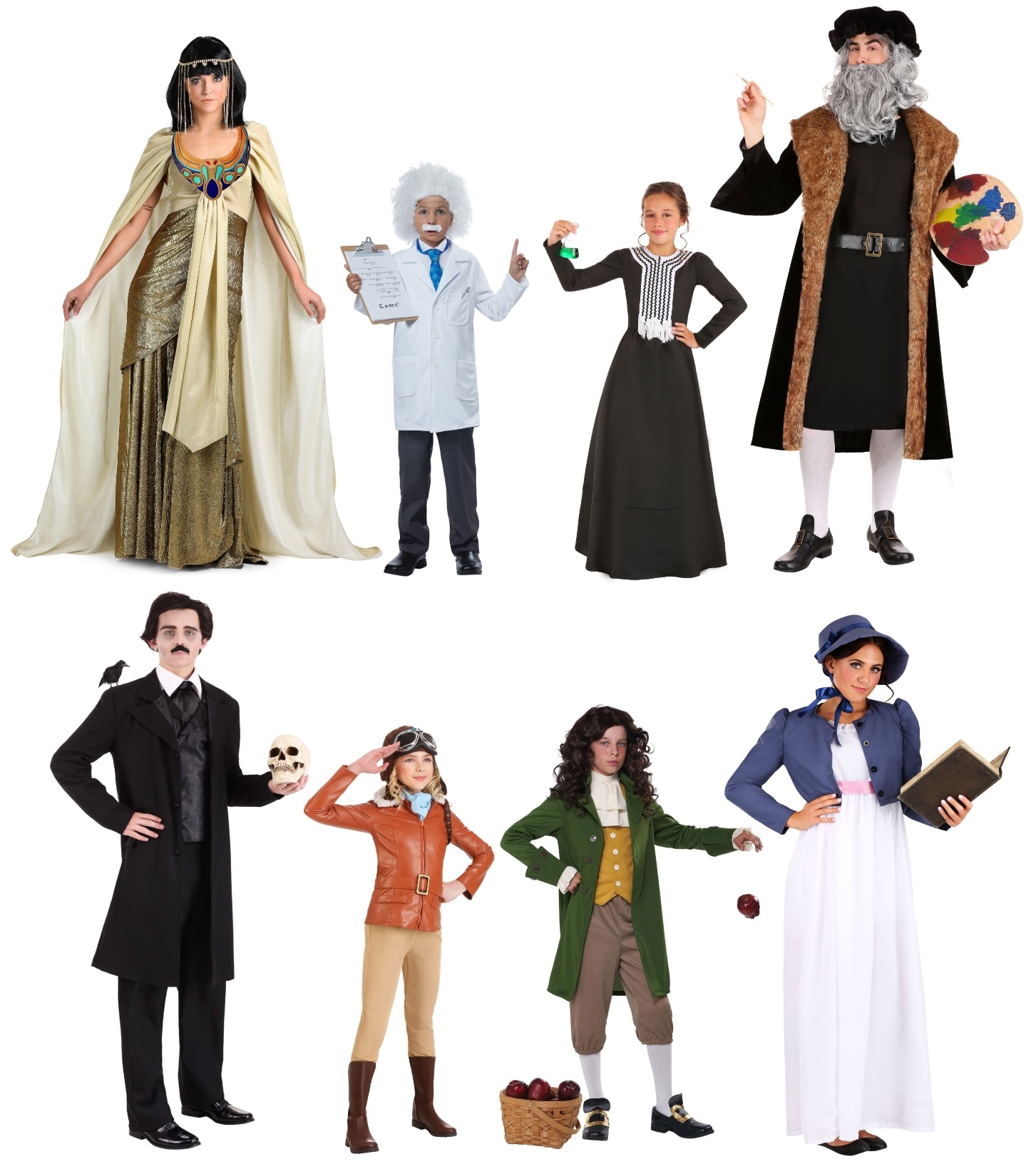The image displays a group of eight people, each dressed in elaborate historical and cultural costumes, suggesting it could be an advertisement for a Halloween costume store. Starting from the top left, a woman is dressed as Cleopatra, complete with black hair, a head wrap, and traditional Egyptian attire. Next to her stands a boy in an Albert Einstein costume, featuring a white lab coat, white poofy hair, and a mustache, with a finger raised and holding a clipboard. Beside him is a girl dressed as Marie Curie in a black dress with white trim, holding a vial of green liquid. To the right, a man portrays Leonardo da Vinci, wearing a black floppy hat, a long black and brown coat, brown shoes, and holding a painter's palette.

On the bottom row, starting from the left, a man dressed as Edgar Allan Poe sports a black suit and holds a skull with a black mustache, complete with a raven on his shoulder. Next to him is a girl dressed as Amelia Earhart, wearing a short blue jacket, a matching hat, and a white gown underneath, alongside a model airplane. A boy dressed as Isaac Newton stands to her right, dropping an apple with a basket of apples at his feet. Finally, a woman dressed in 18th-century clothing holds a book, though her specific identity remains uncertain. This scene effectively captures a diverse array of iconic historical figures, each convincingly represented with detailed costumes.